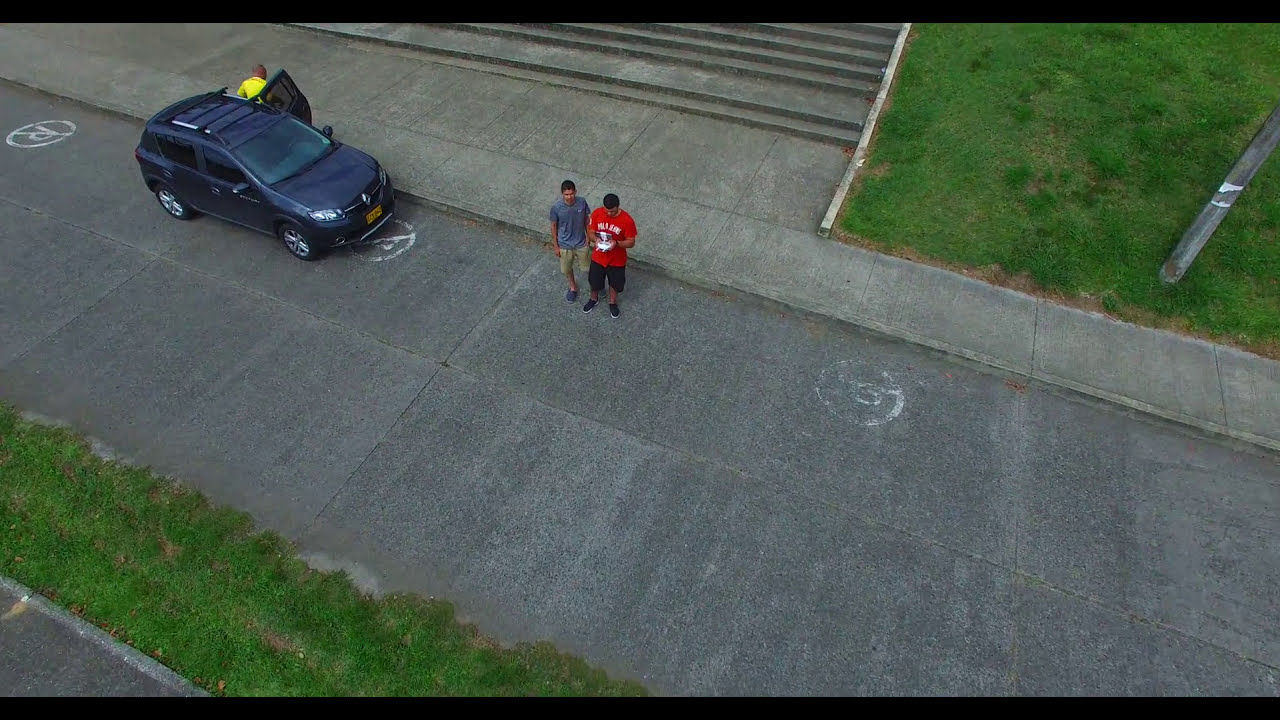The aerial photograph, likely captured by a drone, shows a wide expanse of concrete pavement that runs diagonally from the top left to the bottom right of the image. In the center of the image, two men are standing on the pavement. The man on the right is wearing a red shirt, darker shorts, and dark shoes, possibly holding a drone controller. To his left stands a man in a blue shirt, tan shorts, and dark pants. Painted on the pavement are three white bars, possibly indicating a no-parking zone.

To the upper left corner of the photograph, there is a dark-colored car with its door open. A person in a bright yellow shirt is captured in the process of stepping out of the vehicle. The top right and bottom left corners of the image each feature small patches of green grass, providing a bit of greenery in an otherwise concrete-dominated scene. Behind the two men, there are steps leading to an unseen destination. The photograph appears to have been taken in the late afternoon or early evening, judging by the shadows and lighting.